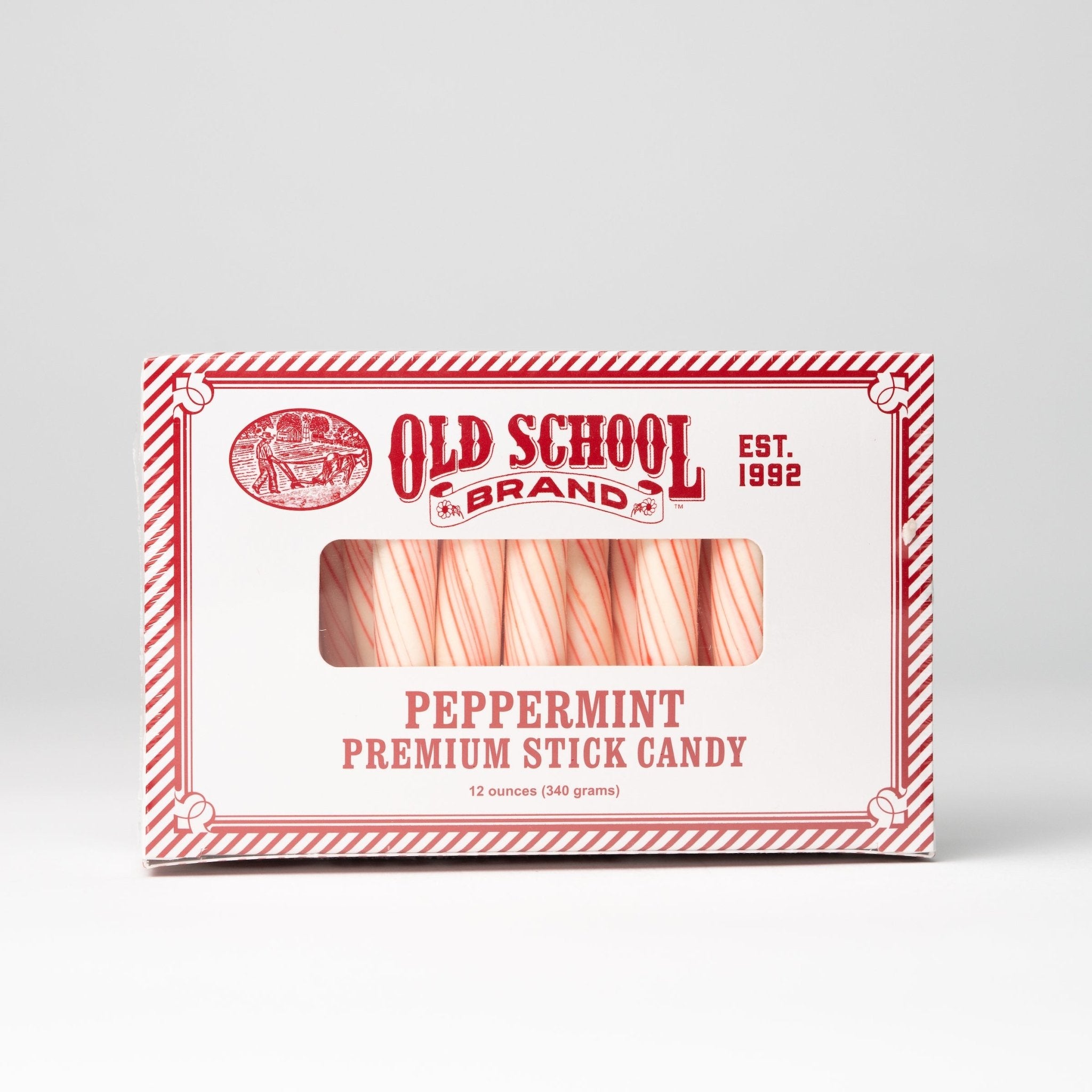This image showcases a box of Old-School Brand Peppermint Premium Stick Candy, established in 1992. The box is predominantly white with red stripes adorning the edges and corners. Centrally, the text reads "Old-School Brand," with "established 1992" displayed prominently to the right. Below, it states "Peppermint Premium Stick Candy," with a weight descriptor mentioning 12 ounces (340 grams). A central plastic window reveals nine thick peppermint sticks, which are mostly white with small red lines. In the upper left-hand corner of the box, there is an illustration of a man plowing a field with a mule, forming part of the company logo. The design is simple yet nostalgic, with a focus on the peppermint motif framing the product.